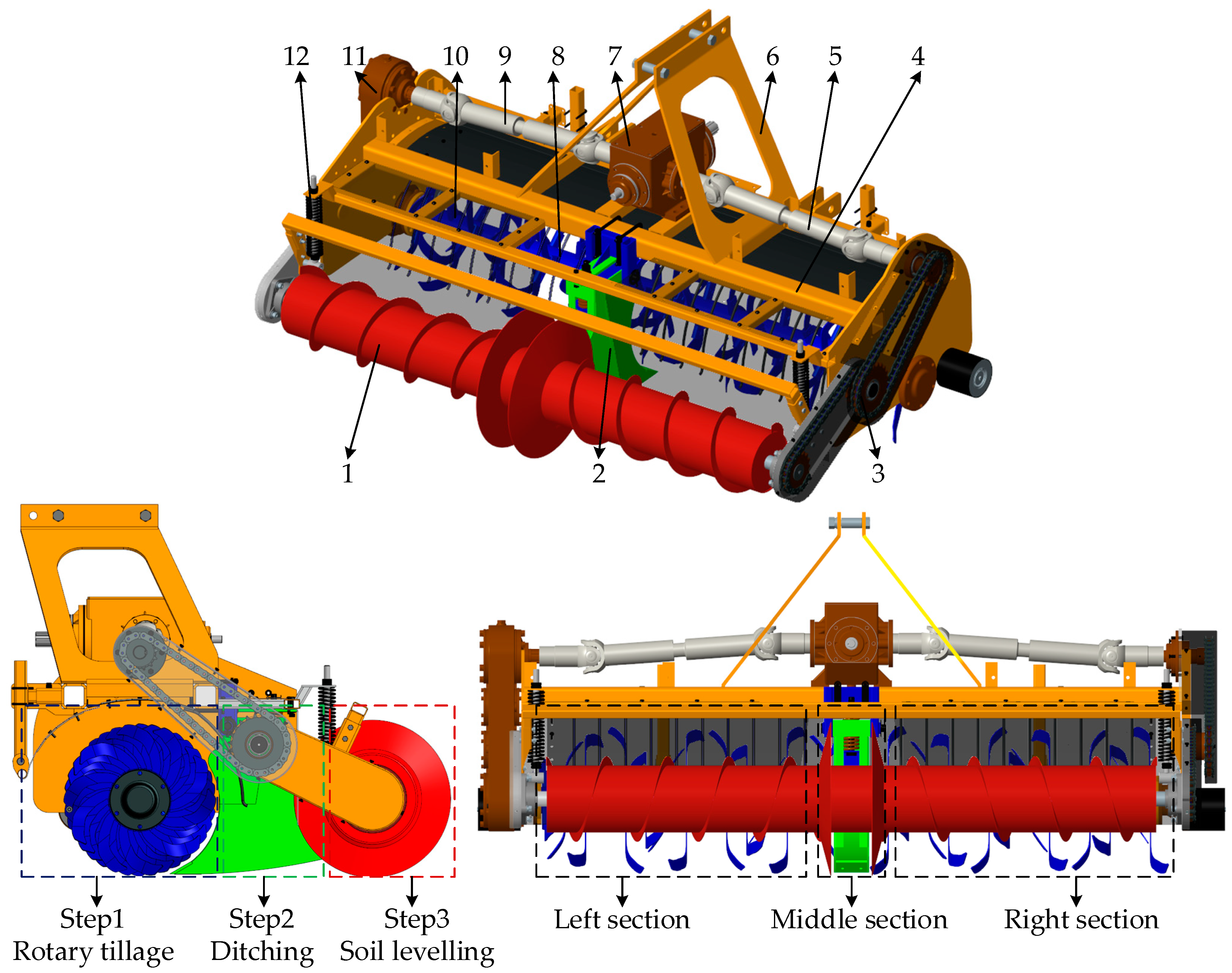This detailed and color-coded schematic diagram depicts an industrial tiller with three distinct viewpoints. At the top of the diagram is a top-down view, highlighting the parallel alignment of the tiller's blades. Below, two images provide different perspectives: the left image presents a profile view of the entire yellow-based tiller, including rotary tillage, ditching, and soil leveling tools in blue, green, and red respectively, while the right image offers a frontal cross-section showcasing the rectangular shape of the equipment and its components. Despite the presence of numbers ranging from 1 to 12 labeling various parts of the tiller, the diagram lacks a legend to define these labels. The use of colors such as blue, green, red, yellow, gray, and brown helps distinguish the different functional segments of the tiller.